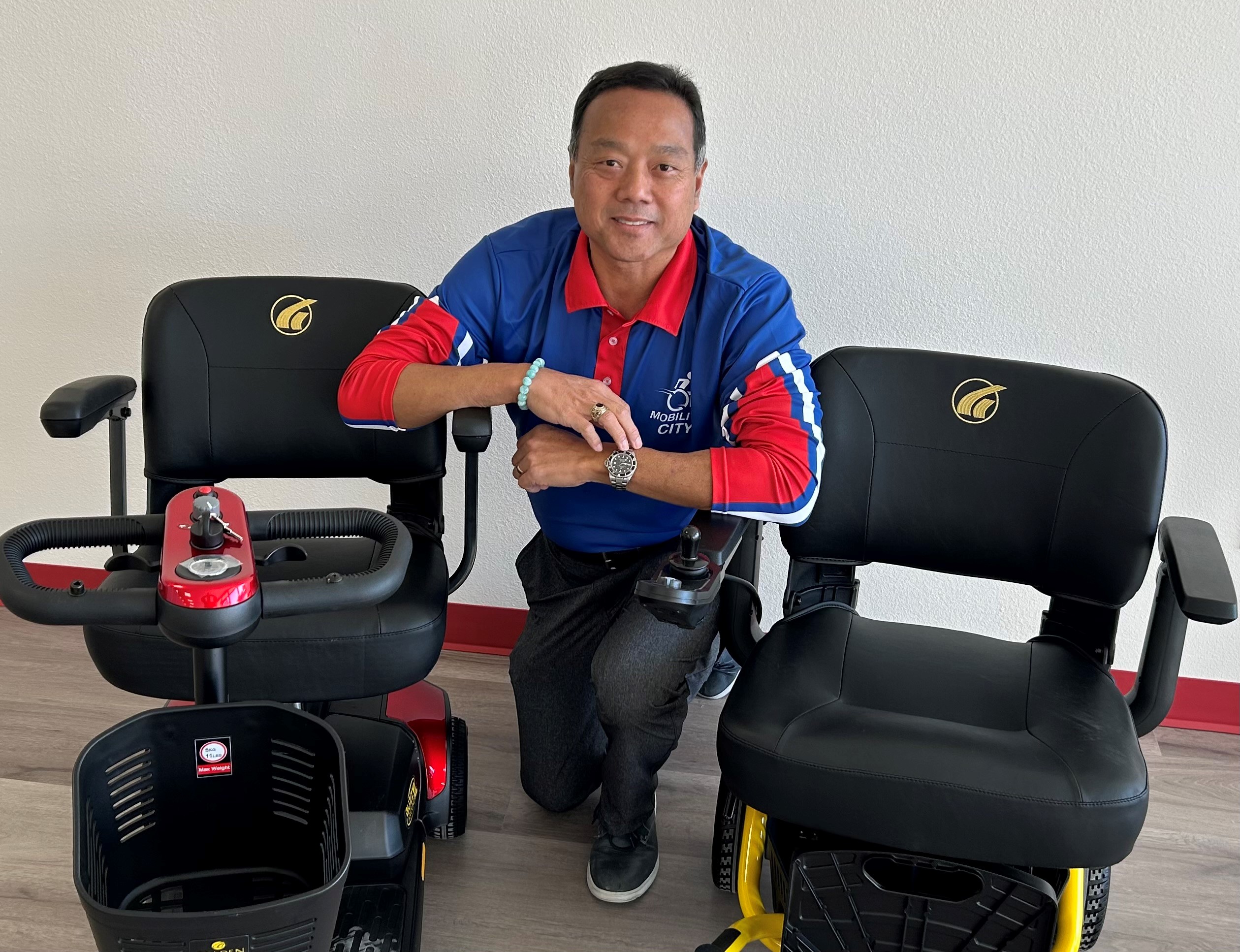In this photograph, an Asian man is kneeling on the ground between two high-tech electronic wheelchairs. He is wearing a red, blue, and white polo-style shirt adorned with buttons on the front. The shirt features a logo near his left chest, depicting a wheelchair with the words "Mobility City" beneath it. Completing his outfit, he is dressed in gray trousers and gray sneakers.

Both wheelchairs have black vinyl cushioned seats and armrests. The wheelchair on the right boasts a bright school bus yellow frame made of tubular metal and is equipped with a joystick positioned on the right armrest for navigation. On his left, the other wheelchair features a unique steering system, with a steering wheel placed at the top for ease of access, accompanied by a red glitter console in the center and a handy black plastic basket attached to the front. The detailed styling and functional aspects of the wheelchairs mark this as a highly specialized and purpose-driven setup.